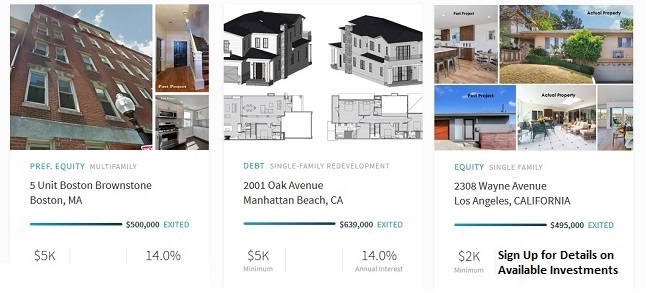The image showcases three property listings:

1. **5-Unit Boston Brownstone, Boston, Massachusetts**: This property is depicted on the left side of the image, showing a tall brick building with numerous windows. Key details include a listing price of $500,000, an edited note to the right, and two statistical figures below - "5K" on the left and "14.0%" on the right.

2. **2001 Oak Avenue, Manhattan Beach, CA**: Positioned on the right side, this listing features two generated images of a house from different angles at the top, with gray blueprints of the interior layout at the bottom. The listing price is $639,000, with "5K" and "14%" noted below.

3. **2308 Wayne Avenue, Los Angeles, California**: Located on the far right, this listing presents five views of the property, one from the outside and four from the inside. The price is $495,000, with "2K" to the left and a prompt to "Sign up for details on available investments" in the bottom right corner against a black background.

All three listings are set against a white background, providing a clean and organized presentation.